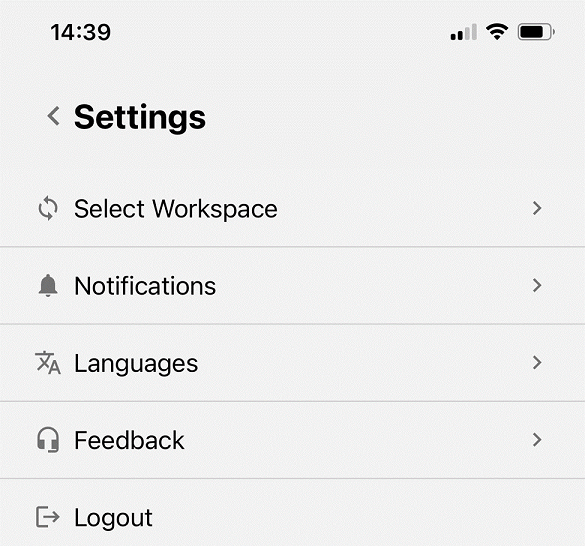This image is a screenshot of the settings page on an Android phone. At the top of the screen, the time is displayed in military format as "14:39". To the right of the time, there is a signal strength icon with four bars, two of which are highlighted, indicating partial signal reception. Adjacent to the signal icon is a fully illuminated Wi-Fi symbol, and further to the right is a battery icon, showing a 75% charge.

Below the status bar, on the left side, there is a gray back arrow. Next to this arrow, the word "Settings" is prominently displayed in bold black font with a capital 'S'. Directly beneath this title is a refresh icon featuring two arrows, depicted in light gray. To the right of this icon, the phrase "Select workspace" is visible, accompanied by a right arrow at the far right.

A horizontal line separates this upper section from the rest of the settings options. The first option features a bell icon with the label "Notifications" to its right, followed by a right arrow. The subsequent entry is marked by a language icon next to the word "Languages" with an accompanying right arrow. The "Feedback" section is next, identified by a headphone icon and a right arrow. Finally, at the bottom of the list is the "Logout" option, distinguished by an arrow icon to its left and a right arrow to its right.